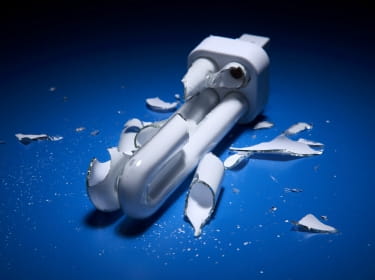In this photograph, a broken light bulb is prominently displayed on a dark blue surface that fades to black at the top edges and corners of the image. The bulb, with a white connector base, consists of two double-looped cylindrical tubes reminiscent of fluorescent light structures. Each tube extends from the base in a U-shape, where the right-hand side tube is partially intact but shattered halfway down. The left-hand side tube is even more thoroughly shattered, with fewer pieces remaining intact. Numerous jagged shards of glass, including a few larger cylindrical pieces, are scattered around the broken bulb. White specks, likely remnants of the shattered light, are also dispersed across the blue surface. This unusual light bulb, not common in typical household lamps, is clearly no longer functional.